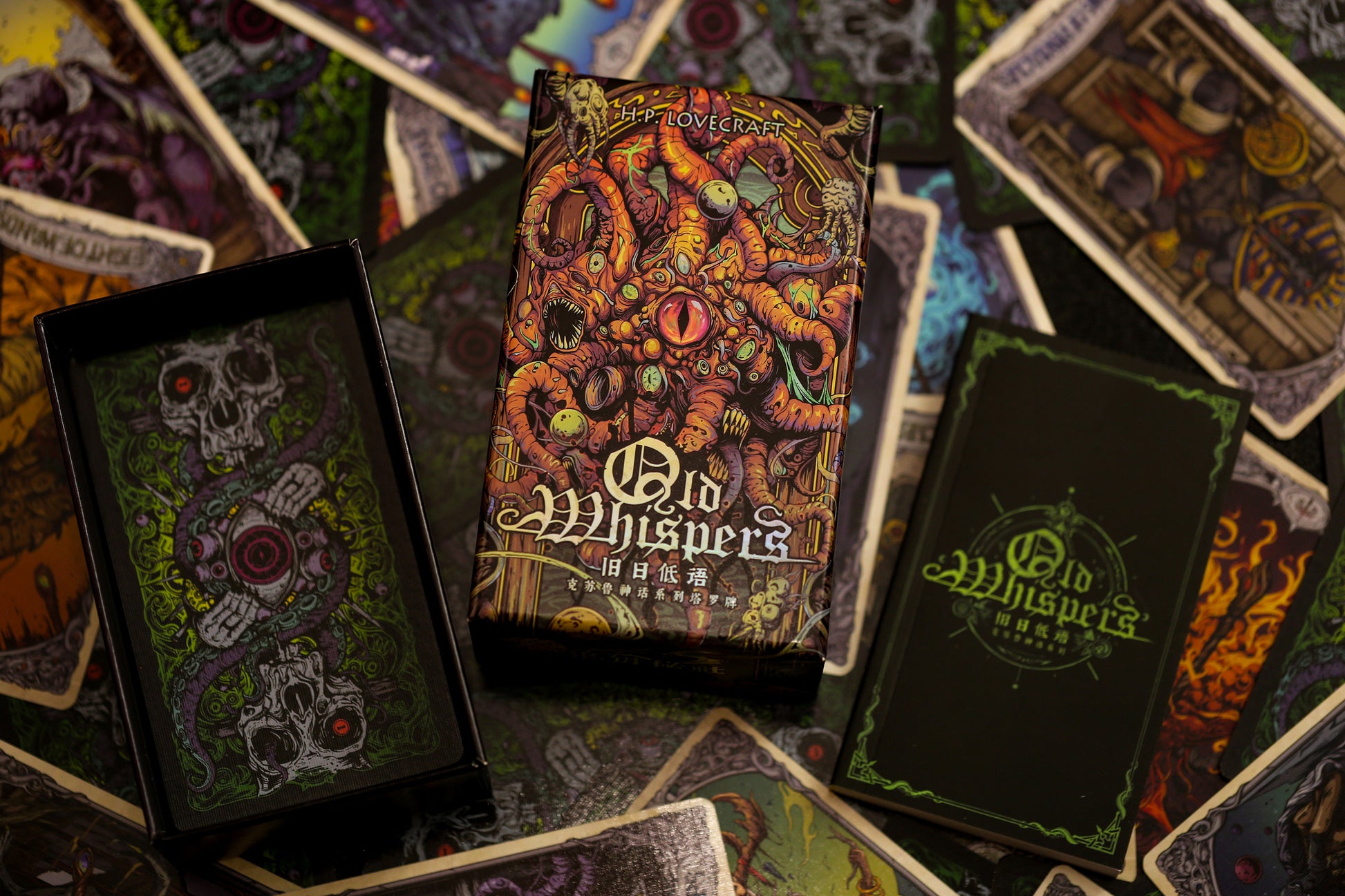The image displays a pile of books with mischievous, eerie-looking covers. At the center of this pile, a book titled "Old Whispers" stands out, slightly turned to the right. The title is written in an orange hue that fades to white towards the bottom, accompanied by Chinese characters underneath. Dominating the cover is a striking illustration of an octopus-like creature, with orange tentacles adorned with green and yellow stripes. Central to this creature is a large, reflective orange eye with a black pupil. The author's name, H.P. Lovecraft, is prominently displayed at the top. 

Adjacent to this central book, in the bottom left corner, is a darker colored book featuring skulls at the top and bottom; each skull has a single red eye. On the bottom right, there's another book with a black cover and a green border. It also bears the title "Old Whispers" and Chinese characters. The rest of the books are piled underneath and around these key ones, but they are blurred and out of focus, contributing to the chaotic and mysterious atmosphere reflected by the distinctive, spine-chilling imagery prominent on the visible covers.